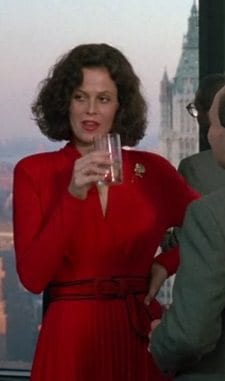The photograph features actress Sigourney Weaver, best known for her role as Ripley in the Alien series. She is elegantly dressed in a form-fitting red dress with a v-neck, complemented by a black and red belt cinching her waist. Her shoulder-length, voluminous brown hair is styled to frame her face as she gazes contemplatively to her right. In her right hand, she holds a clear glass up to her mouth, though the contents are not visible. A gold pin adorns her lapel, adding a touch of sophistication. Sigourney stands poised with her left hand on her hip, positioned in front of a large window. Through the window, a tall, cathedral-like building looms in the misty, gray sky, enhancing the scene's somber ambiance. To her right, there are glimpses of two men dressed in gray suits. One man's shoulder and arm are visible as he gazes at Sigourney with interest, while another man, partially obscured, looks out the window, his eyeglasses catching the light.